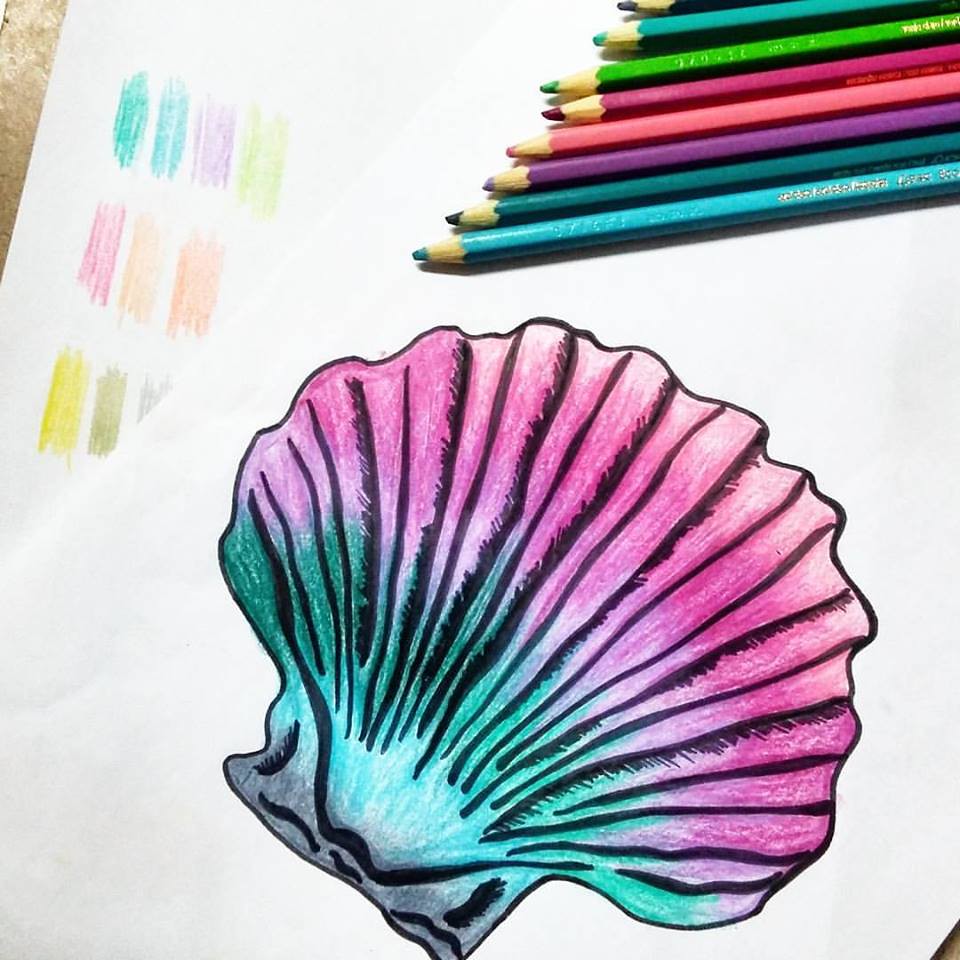This detailed drawing features a seashell prominently centered on a white piece of paper. The shell, meticulously outlined in black, showcases a gradient of colors starting from a light pink on the outer edges, transitioning through shades of darker pink, purple, green, and blue, culminating in a gray hue at the base. The seashell is adorned with distinctive black vertical lines and is slightly tilted to its right side. In the background, another white sheet adds a splash of vibrant color with shades of green, blue, purple, pink, peach, yellow, and green. Positioned above the seashell are a selection of colored pencils in an array of hues, including blue, purple, pink, green, and turquoise, hinting at the lively palette used to breathe life into this captivating artwork.